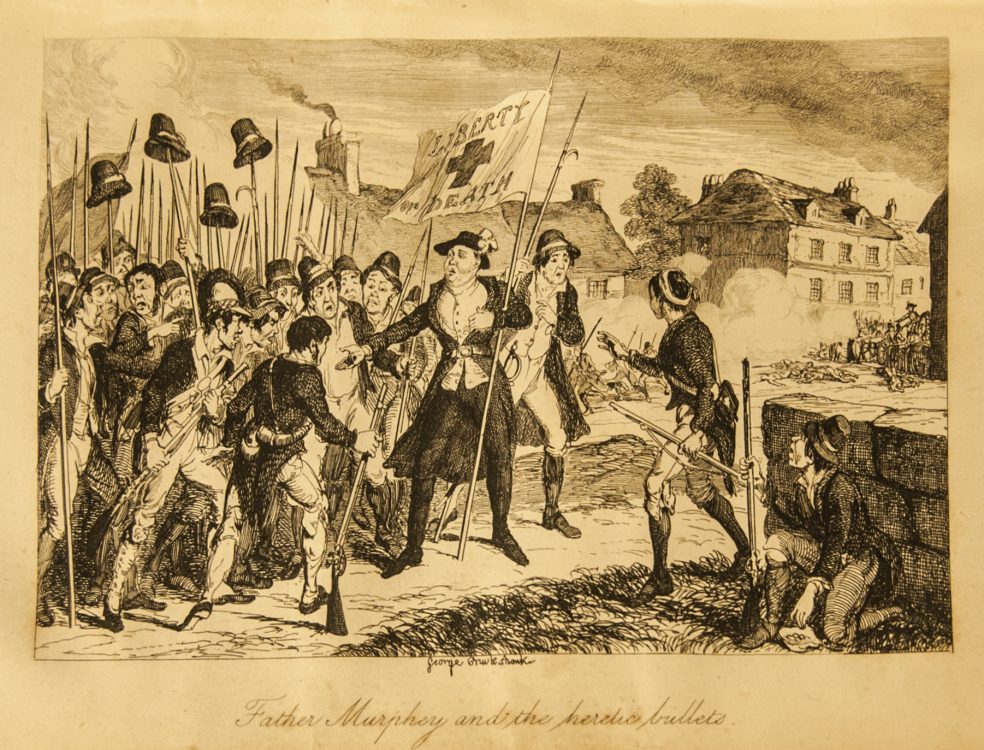This sepia-toned illustration, "Father Murphy and the Heretic Bullets," artistically depicts a fervent scene from the American Revolution. The foreground is dominated by a passionate crowd of men, many of whom are armed with spears adorned with hats. Center stage is a figure raising a flag that defiantly reads "Liberty or Death," adorned with a distinctive red cross. These revolutionaries, clad in long dress coats, tight trousers, and boots, exhibit a range of fervent expressions and stances, with one man notably raising his arms, perhaps rallying the group, while another crouches, surveying the tumult. The scene is set in a war-torn 18th-century town, evident from the historical attire, gunpowder smoke, and cannon fire in the background. Additionally, large houses frame the chaotic tableau, emphasizing the scale of the conflict as the crowd’s fervent spirit contrasts with the burning scene.